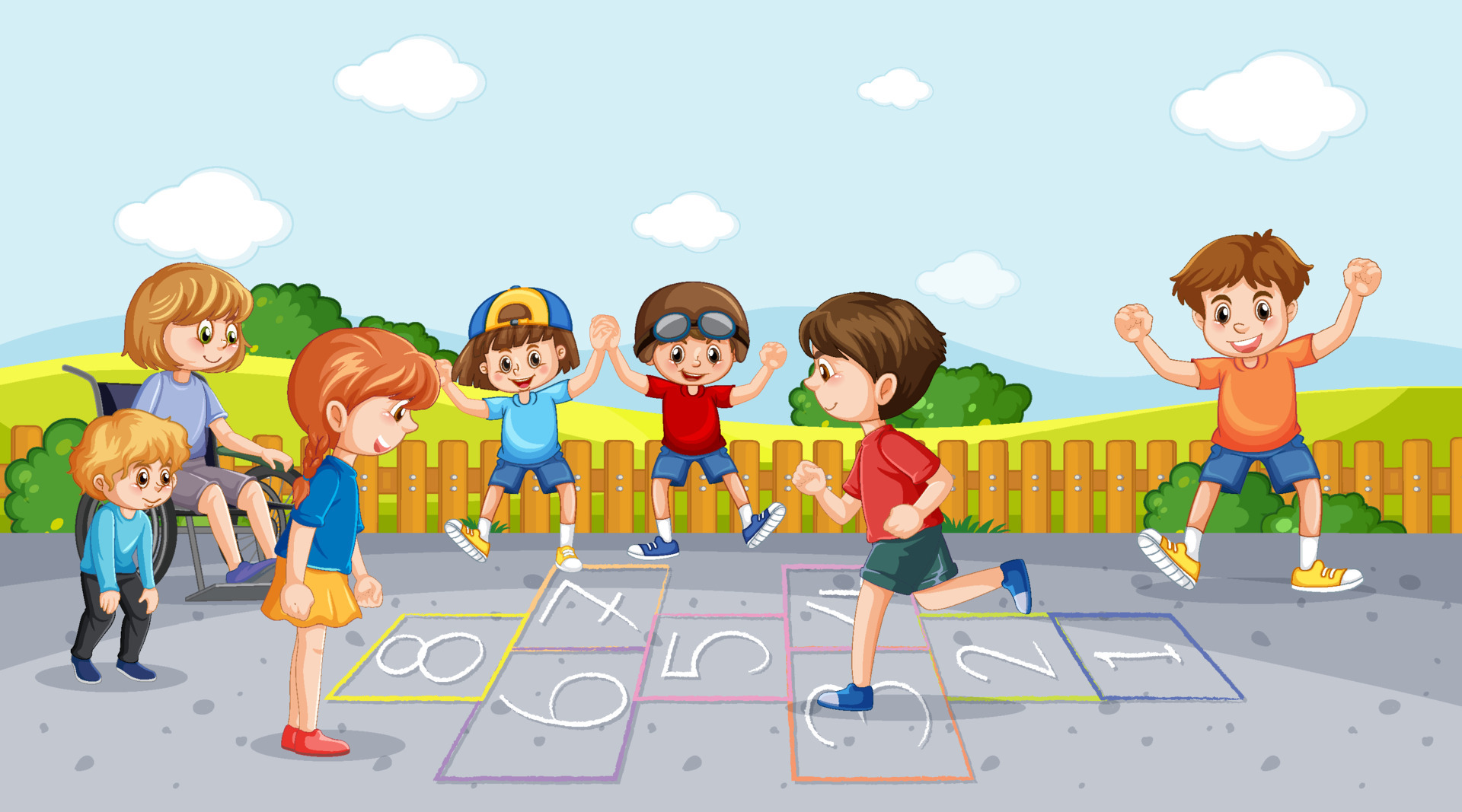The image is a charming, cartoonish illustration of a cheerful schoolyard scene where a diverse group of children are playing hopscotch. The kids, all light-skinned with hair colors ranging from brown to red to blonde, wear a variety of short-sleeved, colorful clothes except for a smaller child on the left in long sleeves. The hopscotch grid, painted in pastel colors with numbers from 1 to 8 in white chalk, is drawn on a tarmac or asphalt ground. One child in a red t-shirt and green shorts is mid-hop on the third square, while another child in an orange t-shirt and blue jean shorts stands on the right with hands raised in excitement. Behind them, two children with headwear—a boy with a blue and yellow cap and another with a cap featuring goggles—are jumping and cheering enthusiastically. A girl in a wheelchair is also part of the scene, observing the game. An older woman stands in the left corner overseeing the activities, with a smaller child next to her. The background is vibrant with a bright blue sky dotted with white clouds, a green rolling hill, bushy trees, and a low wooden fence enclosing the joyful scene.